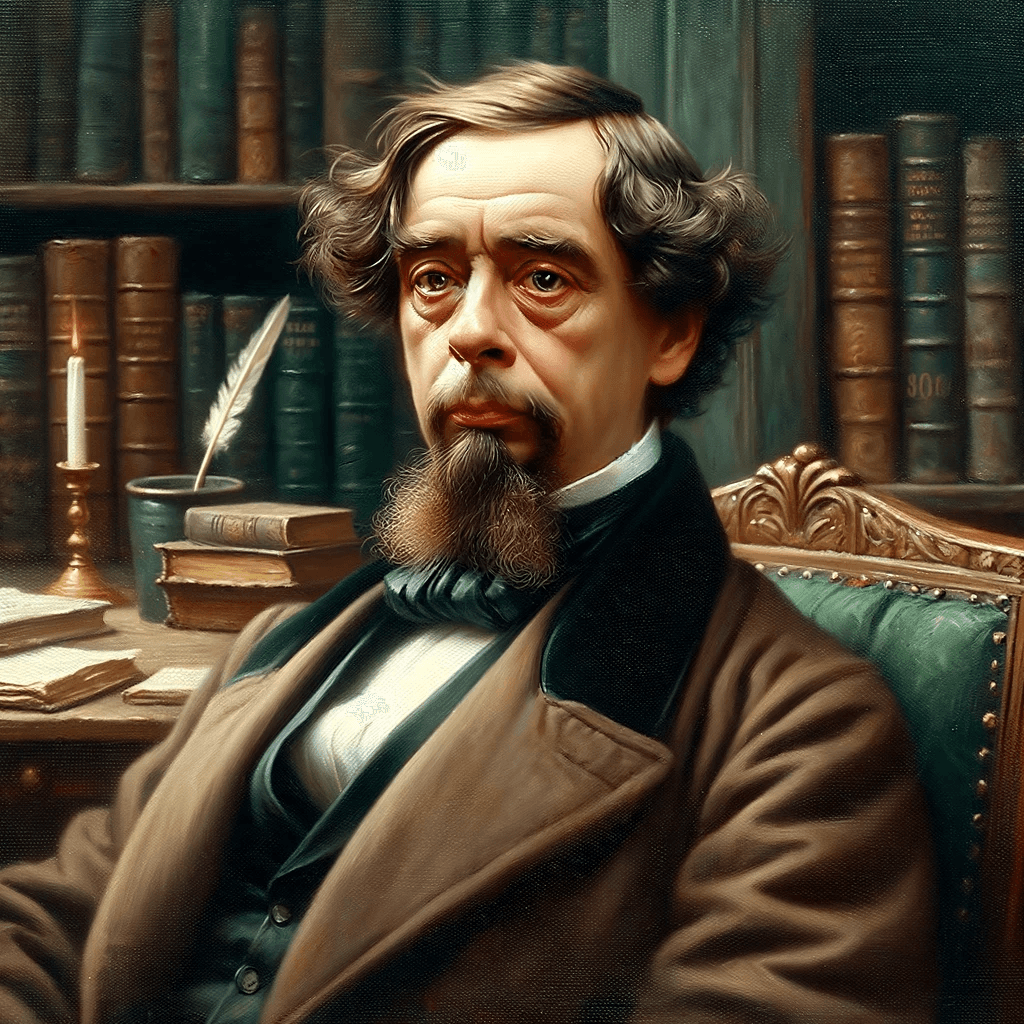A digital art rendering presents a detailed portrait of a middle-aged man, likely in his late 40s, seated in what appears to be a library or study from the late 1800s. The man, possessing a somewhat despairing expression, has a deep crease in his high forehead, bushy eyebrows, and grayish-blue eyes set deeply with noticeable bags underneath. His dark brown hair, parted on the left, is long and curly but does not reach his neck. He sports a prominent mustache and a long goatee.

He is dressed in a brown overcoat with a black leather collar, a bottle green vest, and a white button-up shirt. An elegant scarf completes his attire. The chair he sits on has a wooden frame with green tufted fabric, aligning with his vest.

The backdrop features a collection of old-style, leather-bound books in hues predominantly of blue, green, emerald, tan, and brown, adding to the vintage ambiance. Over the man's right shoulder is a side table or desk holding various items: three stacked books, a candle in a gold candlestick holder, an inkwell with a white feather quill, and several pieces of parchment. The sparse lighting provided by the candle adds a warm, historic glow to the setting. The overall composition highlights both the man's intricate features and the detailed, scholarly environment, evoking a sense of both intellectualism and melancholy.